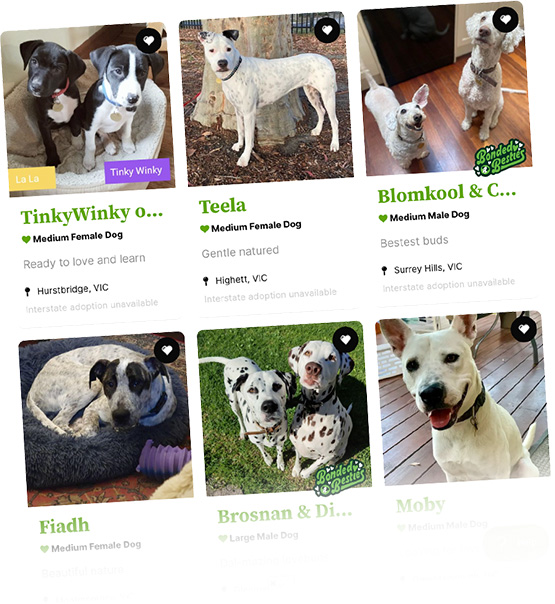The image is a tilted screenshot of an adoption website, showcasing six different breeds of dogs available for adoption. The background of the website is white, and each dog's listing is presented in its own box. The first listing features two puppies named Tinky and Winky, with a location mentioned beneath their image. The second listing shows a white dog named Tila, including details about its size, nature, and location. The third listing displays two white dogs named Blue and Blomkuhl. Following this, the fourth listing is a dog named Fiat. The fifth listing includes two Dalmatians, Bronson and another dog, while the final image is of a white dog named Mobi. Each listing has a small heart icon at the top right corner, allowing users to save their favorite dogs for later. The names of all the dogs are written in green. There is also a watermark on two of the pictures that says "Bonded Besties," indicating that these pairs need to be adopted together.